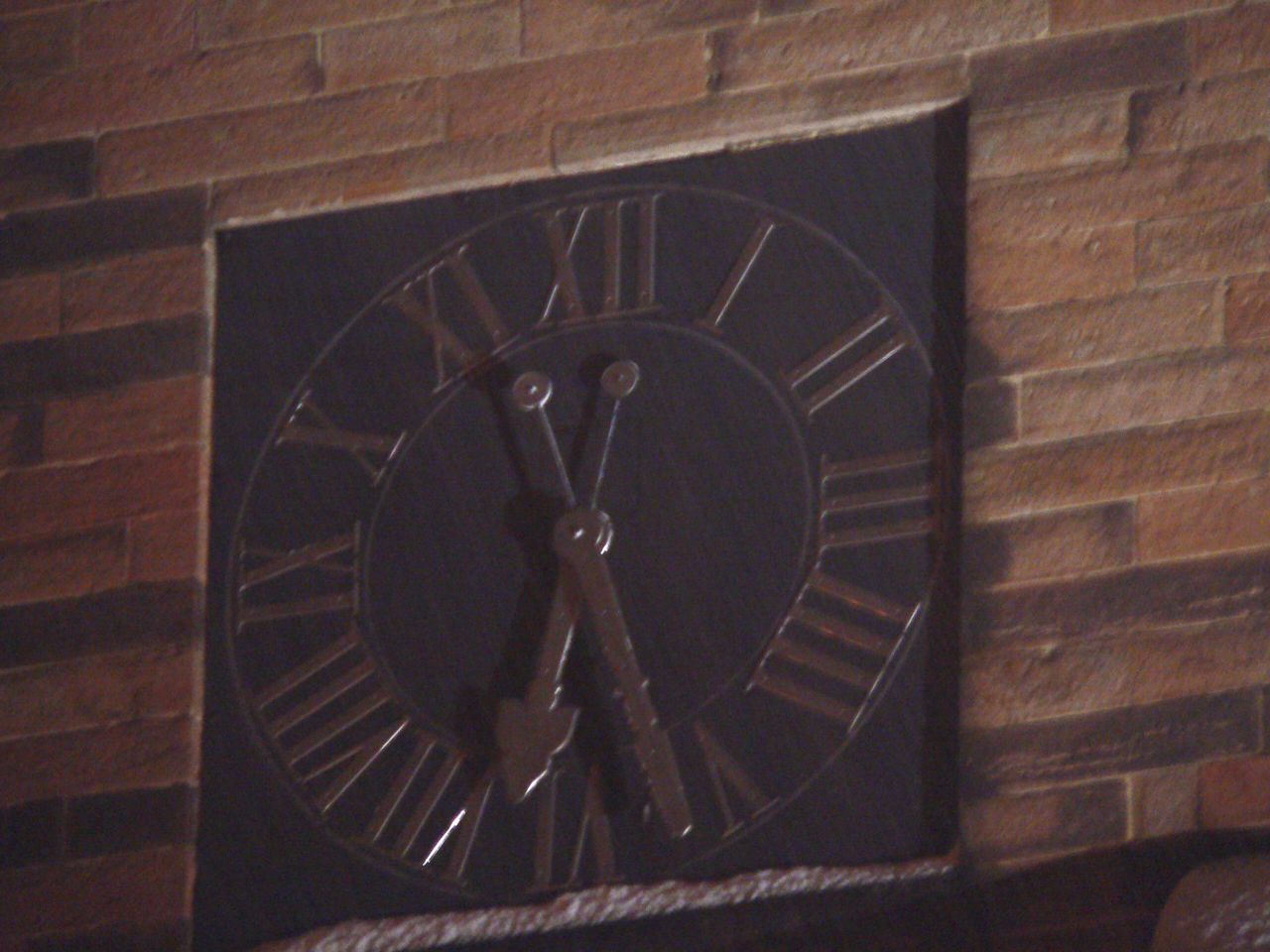In this color photograph, a large, square-shaped, black analog clock with Roman numerals is mounted on a beautifully textured brick wall. The wall exhibits a variety of brick shades, including light brown, dark brown, maroon, and dark gray. The Roman numerals on the clock are bronze-colored, as are the hour and minute hands, which lack a second hand. The time displayed on the clock is approximately 6:27. Below the clock, the brick wall transitions into a dark brown surface. The clock face and hands, both metallic and arrow-shaped, add a striking and elegant contrast to the rustic brick background.